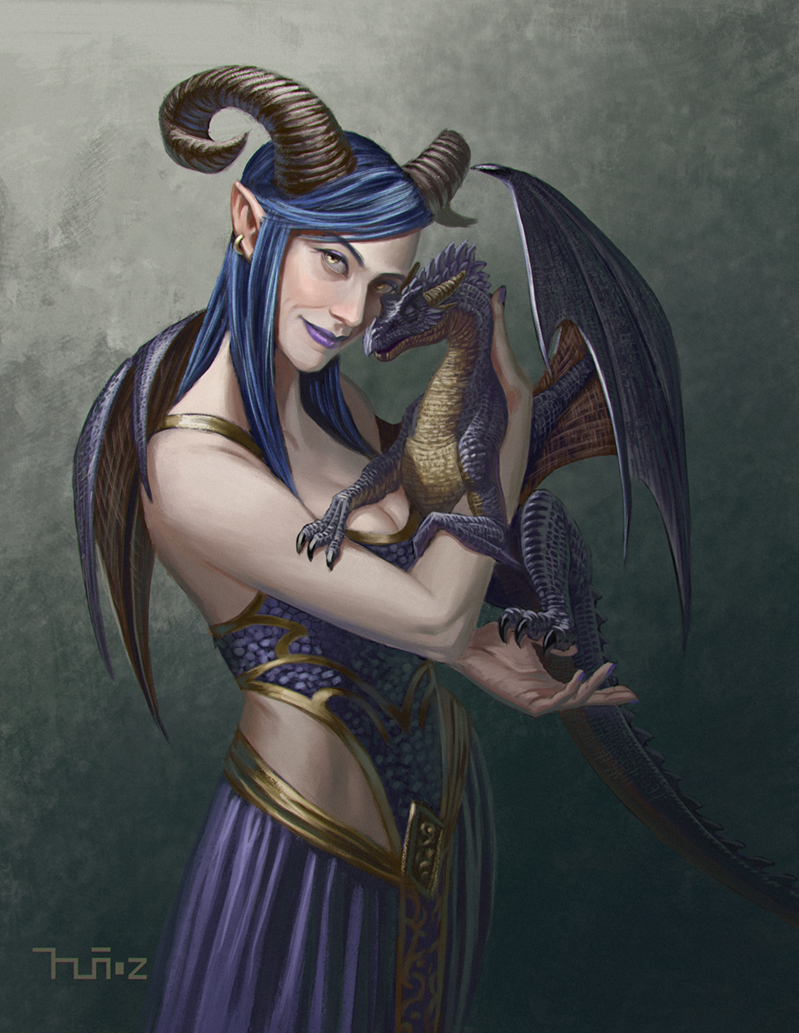The image depicts a fantastical, cartoon-like illustration with an oil painting-like quality, featuring a horned woman holding a small dragon. The woman, who is likely of a white complexion, has unnaturally dark blue hair and a pair of curling ram's horns on her head. Her captivating golden eyes and purple lips add to her ethereal appearance. She wears a revealing purple dress adorned with intricate gold ornamentation and a gold earring, with parts of her arms, hips, and cleavage exposed. 

She cradles a small dragon in her hands, tenderly caressing its face against hers. The dragon, vivid with purplish wings and body, also has a contrasting gold-colored underbelly and some brownish hues on the lower parts of its wings. The entire scene is set against a neutral grey background with subtle lighting variations, primarily brighter in the upper left corner, highlighting the mystical essence of the illustration.